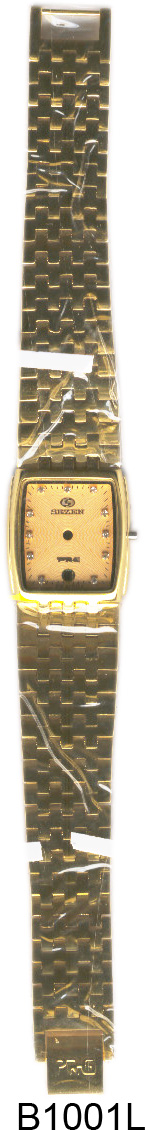The image presents a top-down view of a wristwatch with an open, braided gold metallic strap and silver and gold clasps at each end. The square-faced watch features a gold faceplate, with black markings for the hours and a dial on the right side for adjustments. Despite seeming broken due to light reflections creating the appearance of holes in the gold links, the strap is intact. The watch's face bears the inscription "Cezanne" and has crystal indicators instead of numbers, although the hour and minute hands are faint or missing. At the bottom of the image, the item code "B1001L" is clearly visible in black letters.